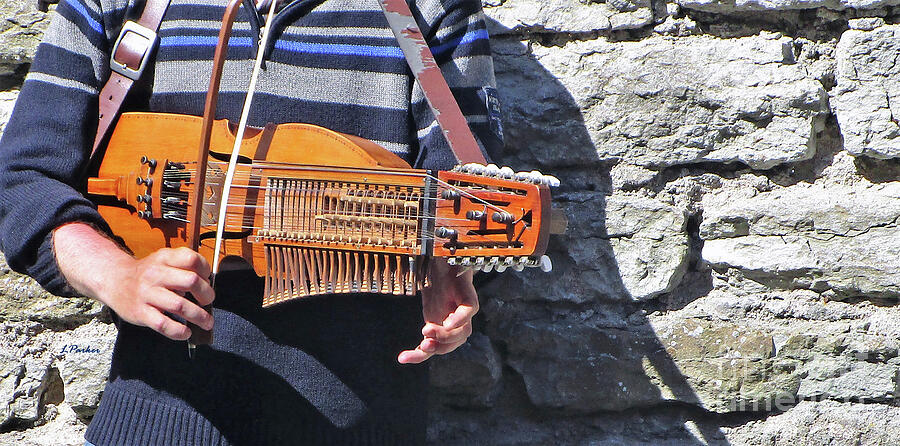This photo captures a partial close-up of an individual standing in an outdoor setting during the daytime, with sunlight casting a shadow. The image focuses on the person's body from the shoulders down to the waist. They are dressed in a striped sweater featuring various shades of blue and gray. The person is holding an unusual musical instrument that resembles a blend between a thick guitar and a violin. This stringed instrument, made of wood and equipped with tuning pegs at the right end and intricate twist mechanisms in the central part, hangs from a leather strap around the person's neck. One of their hands grips the instrument while the other holds a wooden bow, needed to play the instrument akin to a violin. The background reveals a rock wall composed of many stones held together by an older-style mud-cement mixture, adding a rustic touch to the scene.